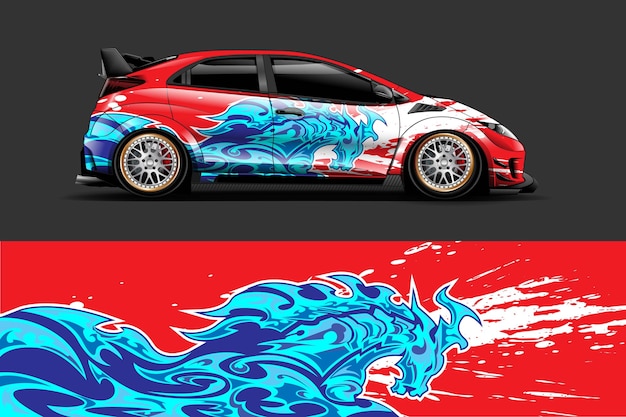The photographic image features two distinct drawings set against an indistinct, likely outdoor background. The upper drawing displays the side view of a small, red, two-door sports car with a sleek and aerodynamic appearance. Prominent features include a bold black spoiler, darkly tinted windows, and gleaming silver hubcaps. A striking, dynamic graphic adorns the side of the car: an electric blue horse in a whimsical, graffiti-like style, galloping with fluid, wave-like motion and exuding energetic vibes, accompanied by white splashes. Below, the second drawing is a close-up of this same blue horse against a red background, highlighting its vigorous and spirited design, contributing to the overall energetic aesthetic of the car. The artistic representation effectively captures the essence of motion and excitement.